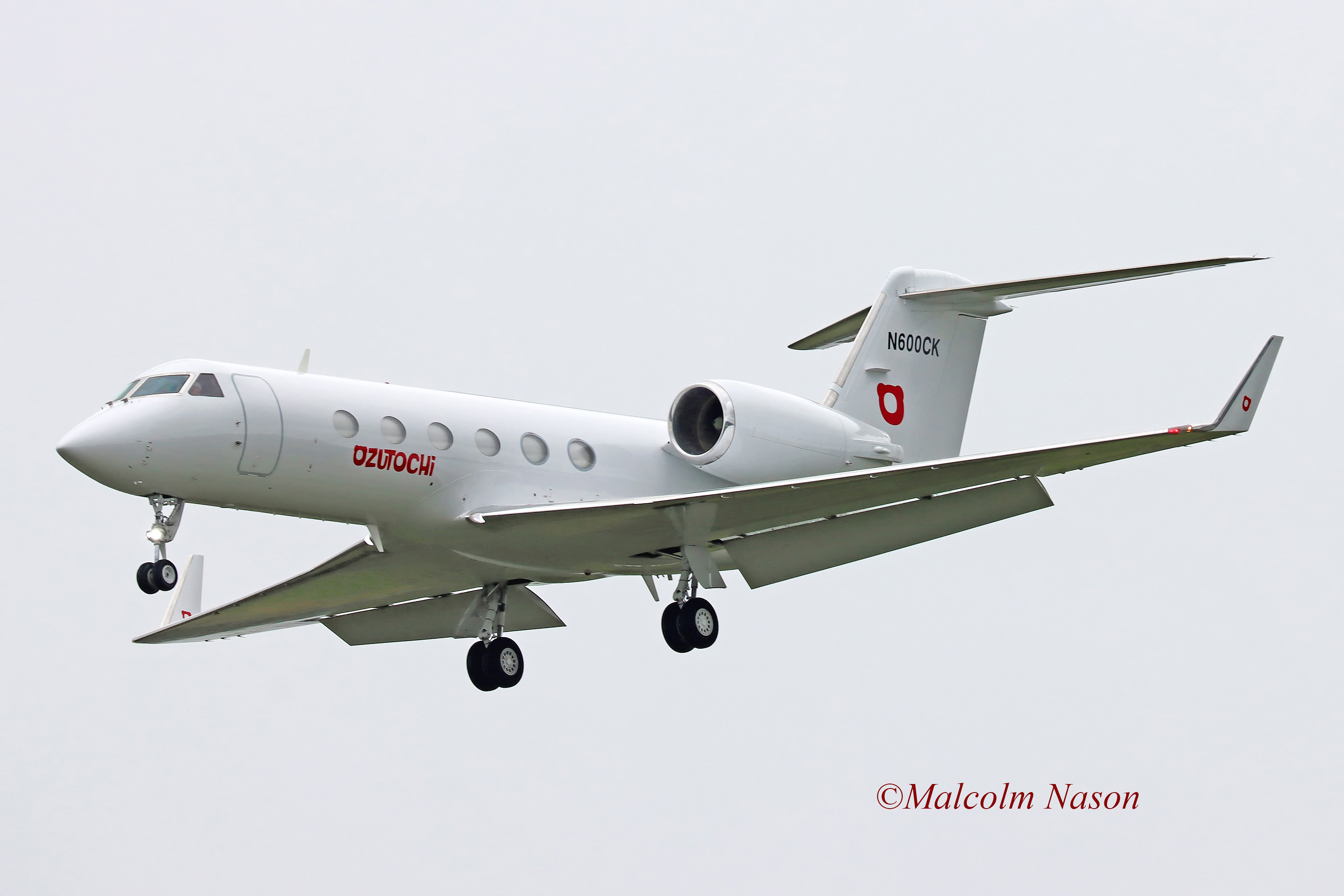In this professional photograph by Malcolm Nason, the centerpiece is a sleek, small aircraft positioned centrally against a predominantly gray background, suggesting an overcast or hazy day. The aircraft, captured in a slightly sideways angle, exhibits a palette of gray, white, red, black, and silver hues, highlighting its streamlined design. The setting appears to be outdoors, possibly at an airport, during daylight hours. The minimalist backdrop emphasizes the aircraft, drawing attention to its details and craftsmanship. The photographer's copyright is subtly present in the bottom right corner, accrediting Malcolm Nason for this meticulous and striking image.